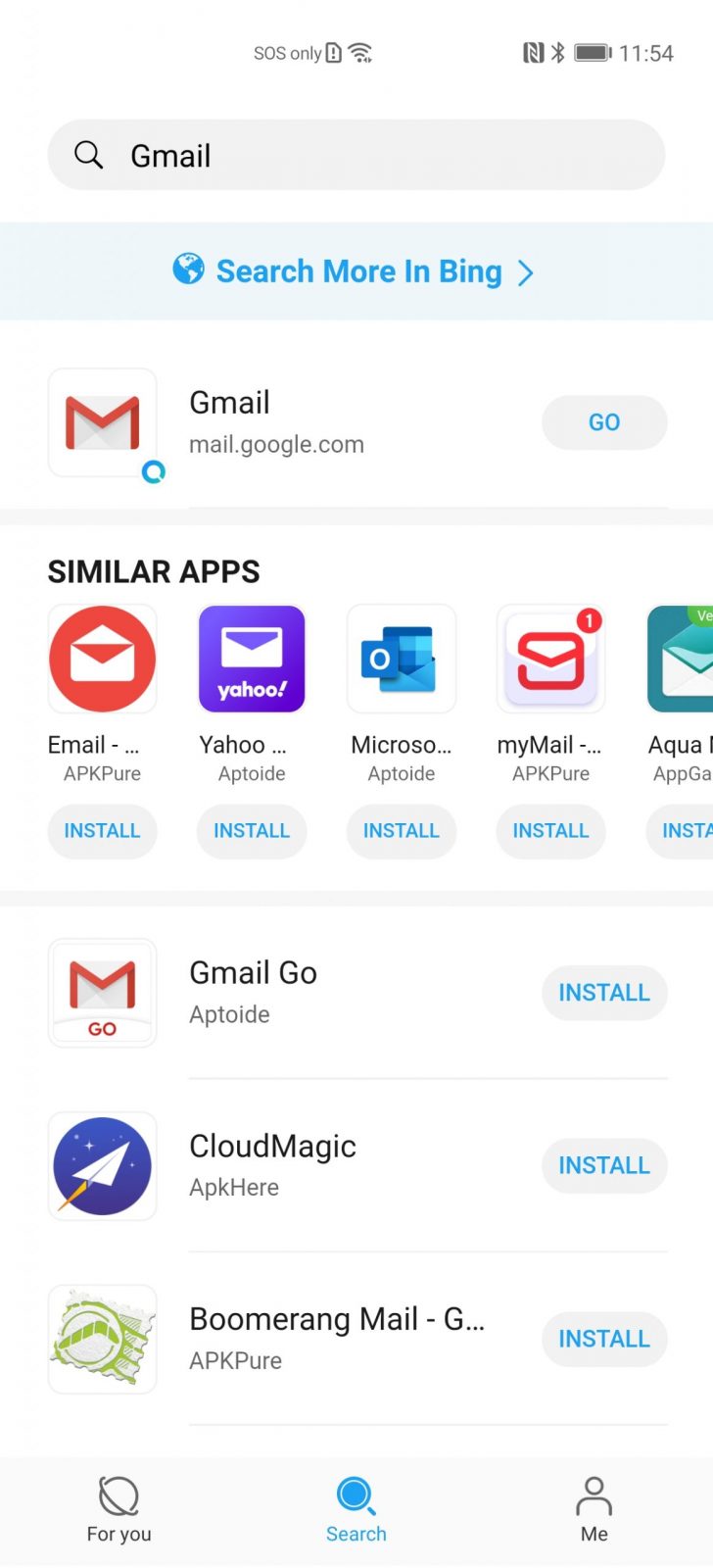In this image, a cell phone's search screen is captured in portrait orientation, perfectly fitting typical smartphone proportions. At the very top, the screen displays “SOS only” indicating limited network availability. Adjacent to this, a fully filled Wi-Fi meter is visible, followed by an icon to the right, a Bluetooth icon, and a nearly full horizontal battery icon. The time displayed is 11:54.

Just beneath these indicators lies a gray search bar with a magnifying glass icon to its left. In black font within this bar appears the text “email”. Below, a small gap of white space separates this from a blue bar in darker blue font, stating “Search more in Bing,” adorned with a globe icon and a right-facing arrow.

Further down, “Gmail” is prominently mentioned next to “mail.google.com,” accompanied by the recognizable Google Mail icon and the text “Go” on its right. The screen then offers suggestions for similar apps, listing “Yahoo,” “Microsoft,” and “MyMail”.

A gray dividing bar underneath separates these suggestions from another section displaying additional app options. The first is “Gmail Go,” featuring a gray install button with blue text and an icon to the right. Following this, “CloudMagic” is presented with the same install button format and an icon showing a blue circle with a rocket ship. The last app listed is “Boomerang Mail,” which also has an install button and an icon resembling a stamp.

At the very bottom of the screen, there are three icons: a globe labeled “For You,” a blue search icon, and a silhouette icon labeled “Me”.